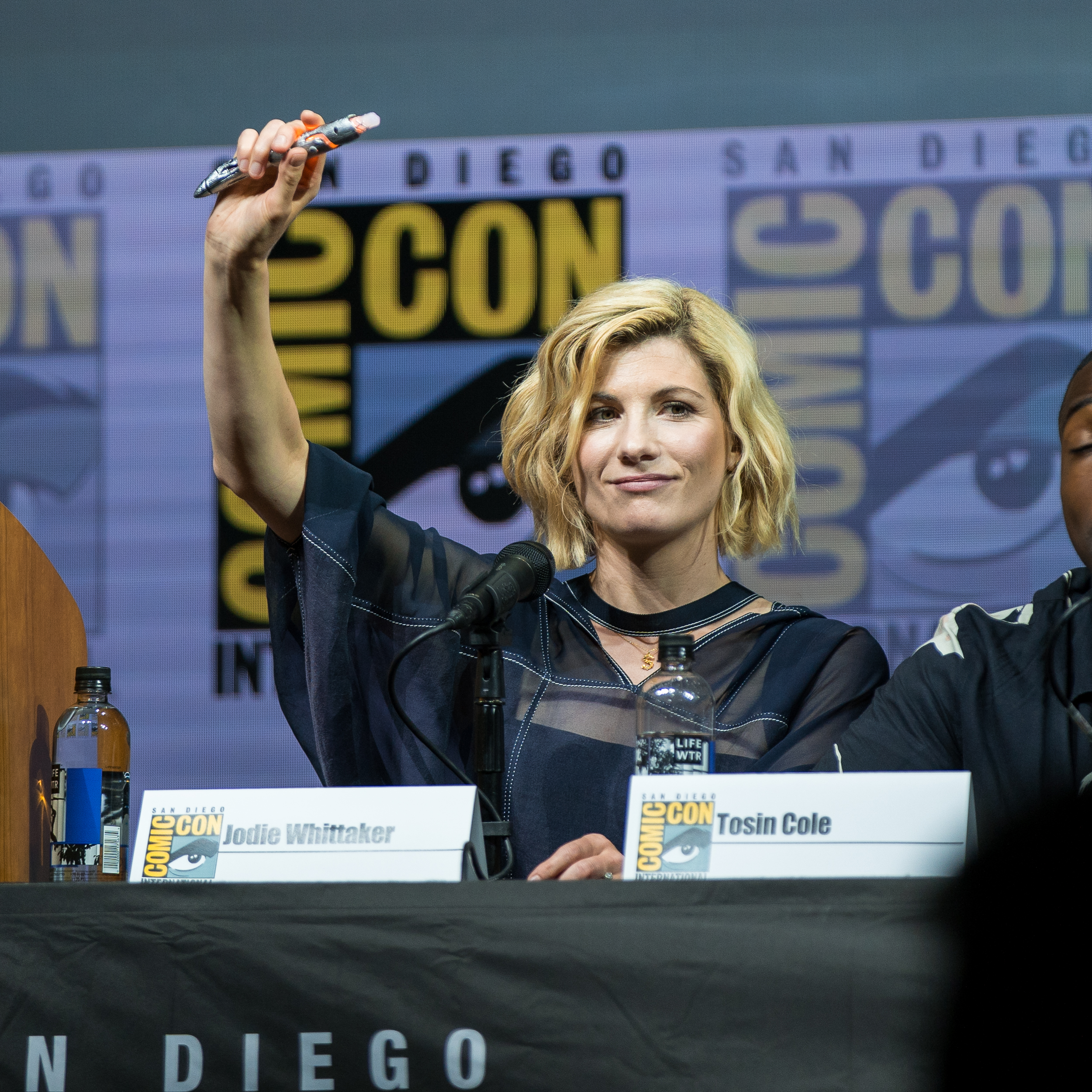The image captures a panel of speakers at Comic-Con San Diego, set against a backdrop that fades from teal-green at the top to a white banner below. This banner prominently displays the words "San Diego" in black letters and features the iconic Comic-Con logo—a black square with "comic" and "con" in yellow letters on opposite sides, and a cartoon eye at its center. In the foreground, a black table with "Diego" written in white letters rests before the panelists. 

Among the three speakers at the table, the most visible is Jodie Whittaker, who famously portrayed the female Doctor Who. Whittaker, with short, wavy blonde hair, dons a black outfit and is seated behind a white name tent that reads "Jodie Whittaker." She has one arm raised, holding what appears to be a pen with a gold or silver body and orange accents. A couple of water bottles and a microphone are also positioned nearby on the table. Whittaker’s expression is engaging, her gaze directed to the right, hinting at a clever and thoughtful demeanor.